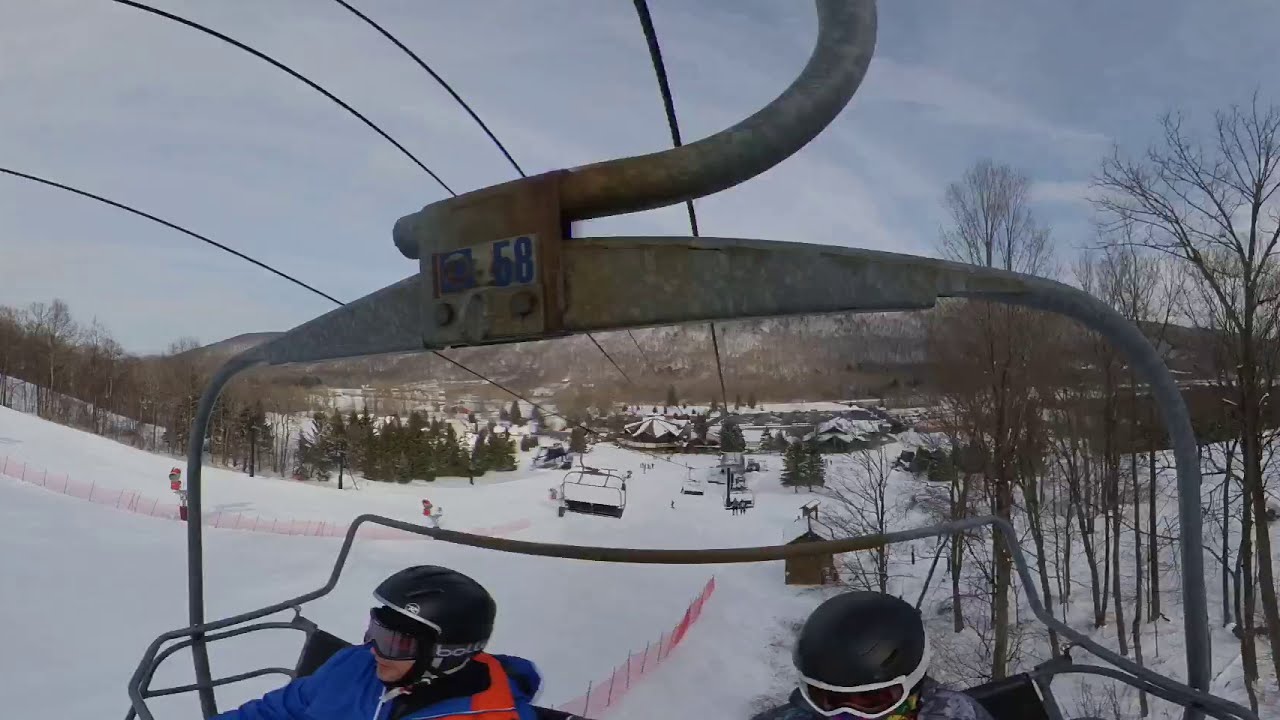This detailed outdoor photograph captures a scenic ski lift experience on a snow-covered mountain. Taken from behind the occupants of a ski lift chair, the vantage point shows two skiers sitting side by side, ascending the mountainside. The skier on the left sports a black ski helmet and goggles, complemented by a blue and orange jacket. The skier on the right also dons a black helmet and ski goggles with white trim, though their clothing is partially cut off by the bottom edge of the frame. Behind them, another ski lift chair, carrying two more skiers, moves upward against the backdrop of rugged mountains and a crisp, blue sky interspersed with white, wispy clouds. Red stripes marking the ski run streak down beneath the lift, adding a vibrant contrast to the serene winter landscape. To the left, a dense cluster of leafless trees, resembling Christmas trees, ascends alongside the lift, while a smaller group of trees lines the right side of the photo. The overall scene conveys a sense of adventure and tranquility, framed by nature's winter beauty.